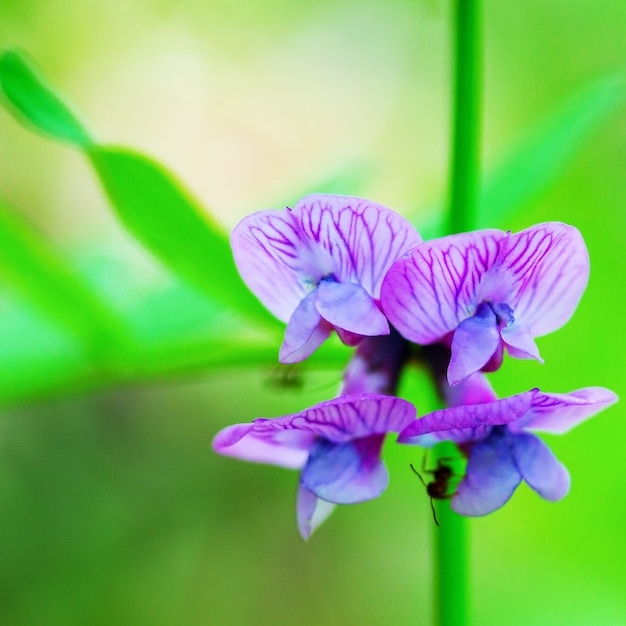This is a highly detailed, close-up photograph of a cluster of flowers resembling orchids, potentially Lady Slippers, displaying a stunning range of purple hues. The flowers have four prominent petals, each adorned with intricate dark purple veins that traverse their lighter purple surfaces, at times fading into white. In the center of these blooms, there are two distinctive pepper-shaped structures and a darker central element.

A particular point of interest is the bottom right petal, where a small, red ant is precariously perched. Although the ant itself is blurry and its precise details are hard to discern, its antennae, body segments—including head, thorax, and rear—and multiple legs can be vaguely made out.

The background of the image features green stems and leaves, partially lit by sunlight, rendering a washed-out or smudged green that accentuates the crisp focus on the flowers in the foreground.